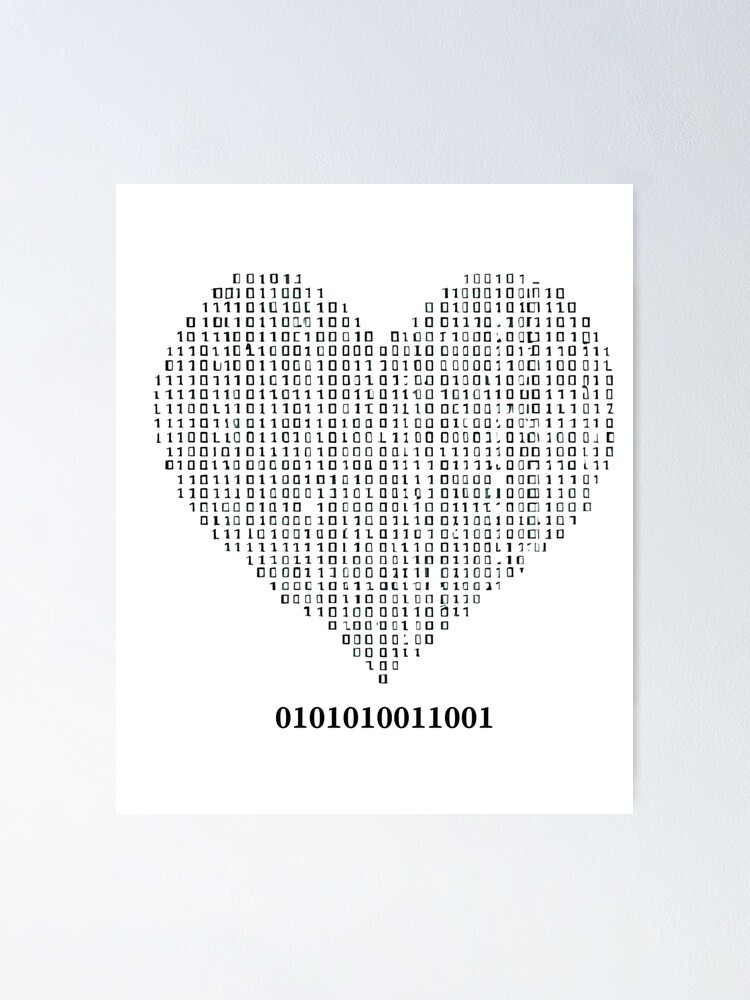The image features a heart composed entirely of binary code (ones and zeros), set against a white rectangular background. This backdrop is placed on a larger, diagonally fading gray background, with the right side appearing quite gray and transitioning to an almost white bottom left corner. Beneath the heart, bold black text displays the binary sequence "0101010011001." The heart, in standard black text, is potentially indicative of a hidden or secret love-related message encoded in binary.